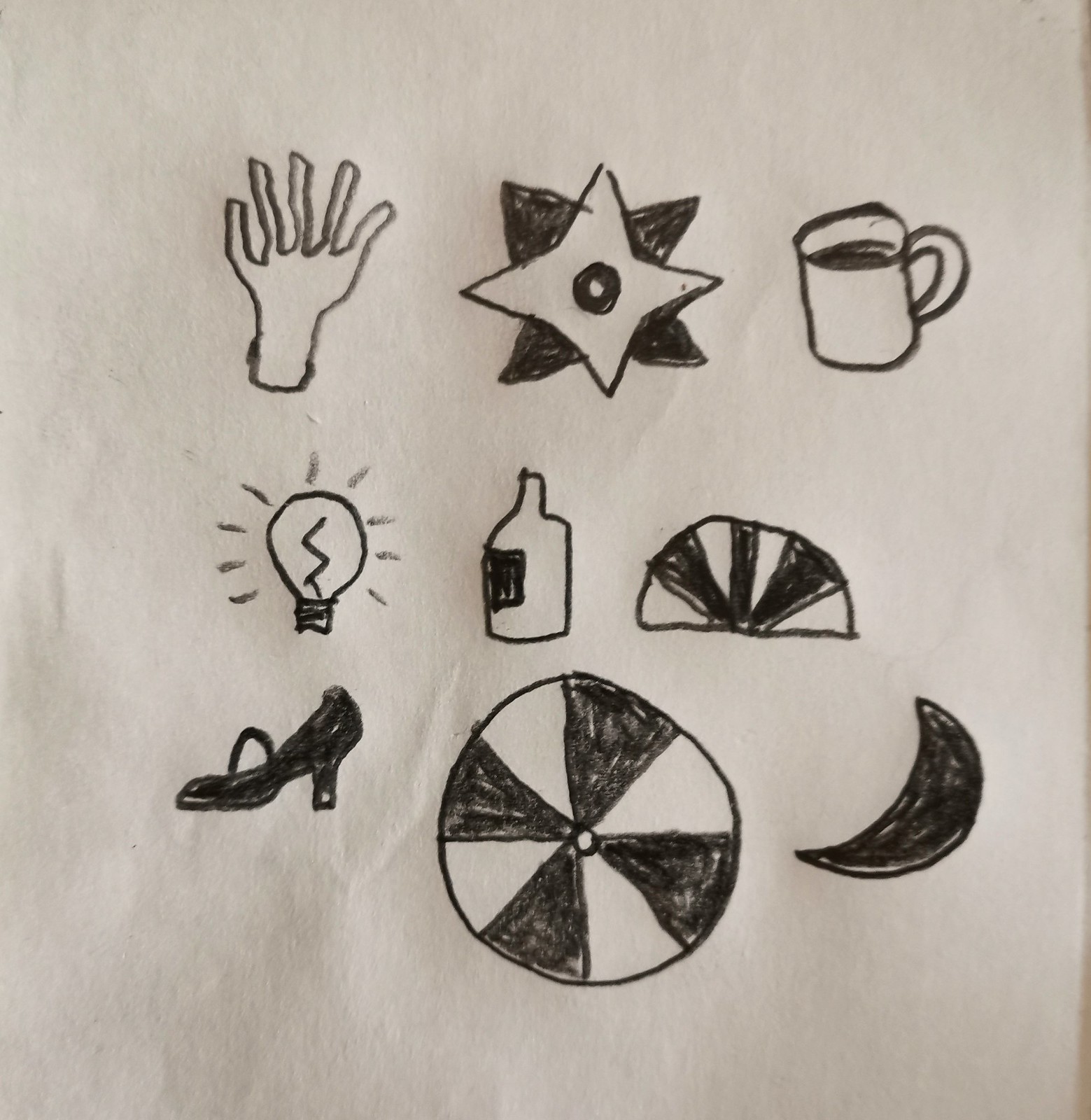The image is a roughly square, off-white bar napkin featuring a detailed black pen or marker collage arranged in a three-by-three grid. Each square contains a distinct, meticulously drawn item:

- **Top row (left to right):** A hand with long fingers, a star shape with multiple points (one white and one black), and a coffee mug with a handle.
- **Middle row (left to right):** A glowing light bulb with rays emanating, a jug or bottle with a black label, and a half-circle with vertical black and white stripes.
- **Bottom row (left to right):** A high-heeled woman's shoe, a circle with black and white wedge-shaped segments, resembling a spinning wheel, and a black-colored crescent moon pointing left.

These distinct and intricate drawings, primarily executed in black, form an eclectic and visually engaging collection of everyday objects and symbols.